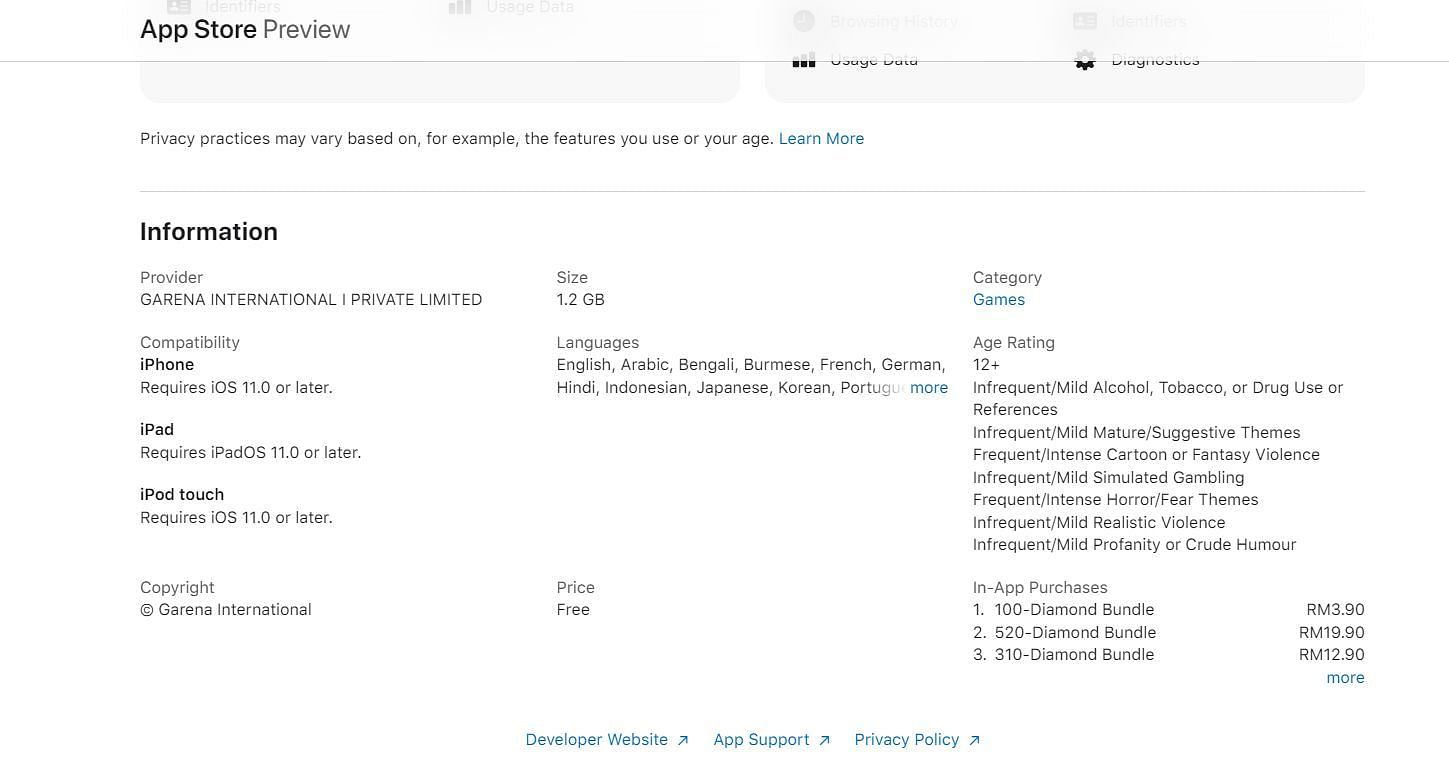The image depicts a section of the App Store preview page with a prominent gray box at the top, partially obscuring some underlying text. Below the gray box is a statement in fine print: "Privacy practices may vary, for example, based on the features you use or your age." A blue hyperlink labeled "Learn More" follows this statement. Directly beneath, on the left side, there's a segment providing information about the app's provider, reading: "Information Provider: Garena International Private Limited." Below this, the compatibility requirements are listed: "iPhone requires iOS 11.0 or later; iPad requires iPadOS 11.0 or later; iPod touch requires iOS 11.0 or later." Copyright information for Garena International is also provided.

In the middle column, details include the app's size, "1.2 GB," and supported languages, which are English, Arabic, Bengali, Burmese, French, German, Hindi, Indonesian, Japanese, Korean, and Portuguese. The price of the app is indicated as "Free," and it falls under the category "Games." Additionally, the section mentions the age rating for the app, though the actual rating is not visible in the provided description.